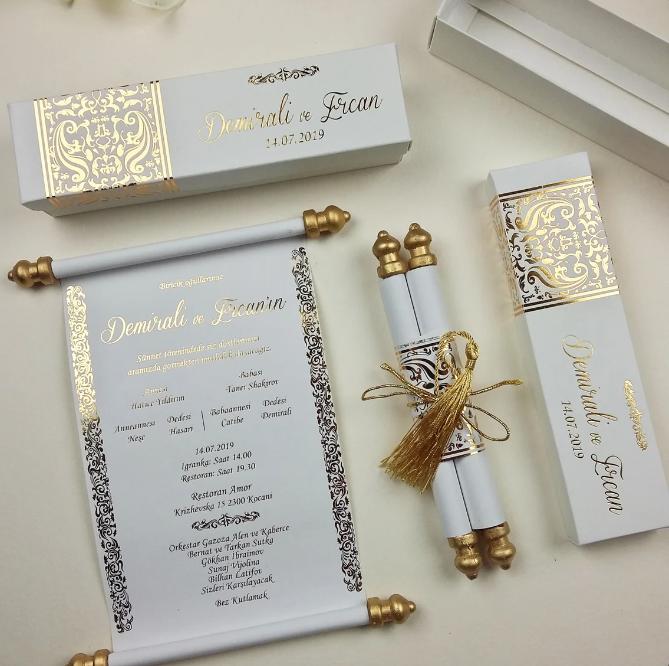The photograph depicts an exquisite wedding invitation set, artfully displayed on an off-white background. The centerpiece is an open scroll with elegant gold text, featuring the names "Demirelli" and "Freon," and the date "14-07-2019." Gold symbols adorn the sides of the scroll, whose top and bottom margins are white, while the ends are accented with gold. Along with the open scroll, there is a closed scroll tied elegantly with a gold ribbon and tassels.

Two white rectangular boxes, both adorned with intricate gold and silver patterns, are part of the set. Each box bears a gold emblem above the names "Demirelli vs. Freon," aligning with the details on the scrolls. The smaller text on the open scroll, likely outlining the event's program or details, is difficult to read due to its fine gold print and glossy finish. This sophisticated ensemble suggests a modern take on the traditional scroll, crafted to announce the joyous occasion of a wedding.